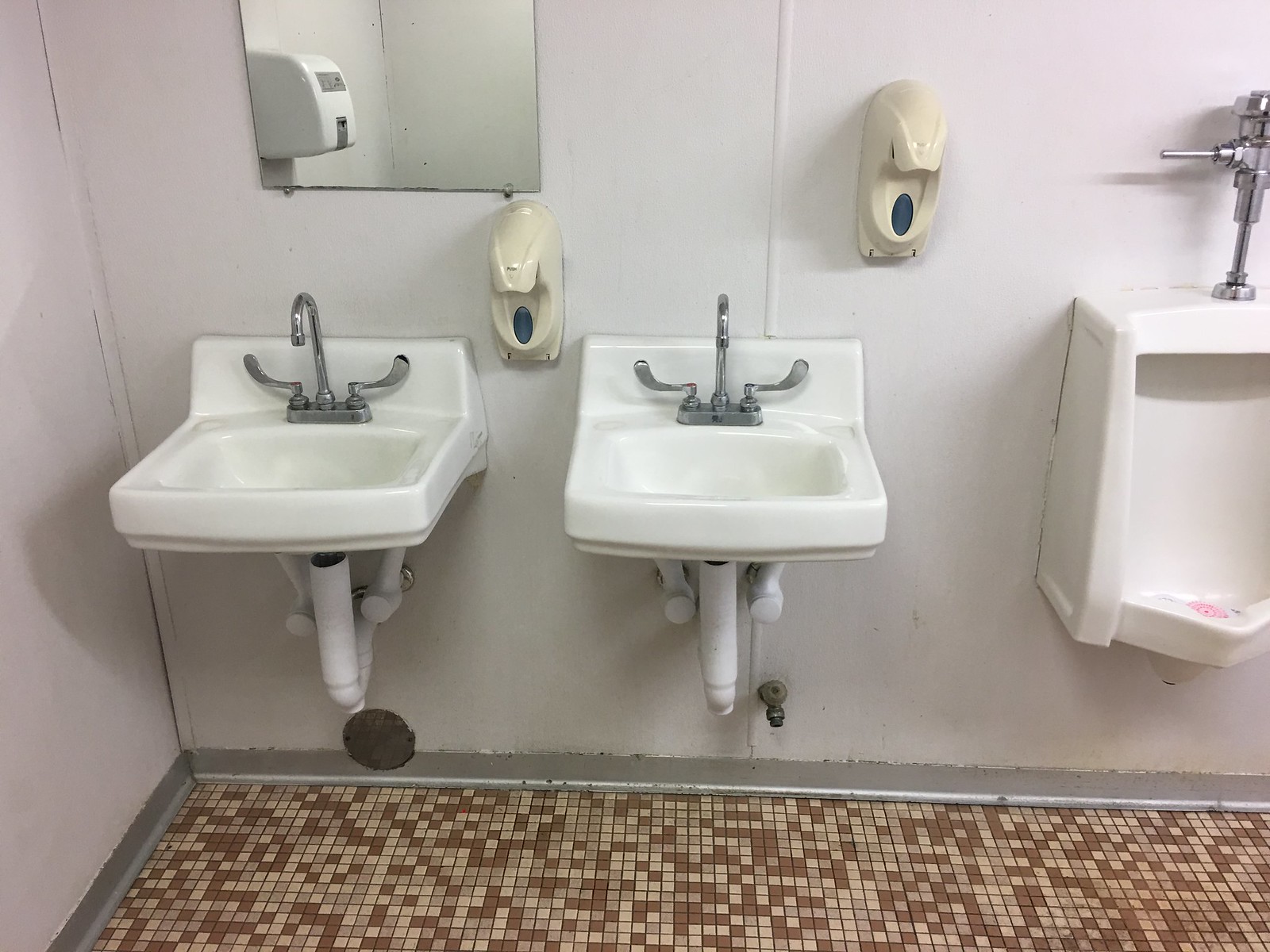This image depicts the interior of a men's restroom with pale, white-ish walls that have a subtle pinkish cast. The floor is covered in small, inch-square tiles arranged in shades of brown, beige, and cream, bordered by a gray rubberized trim. The restroom features two wall-mounted sinks, each fitted with white coverings over the pipes and single-spouted, double-handled faucets. There are two soap dispensers: one positioned between the sinks and another higher up on the wall to the right of the second sink. Above the sink in the corner is a mirror, reflecting part of the side wall and a paper towel dispenser. Adjacent to the sinks is a urinal with a handle at the top and a deodorant cake at the bottom, confirming the setting as a men's restroom.